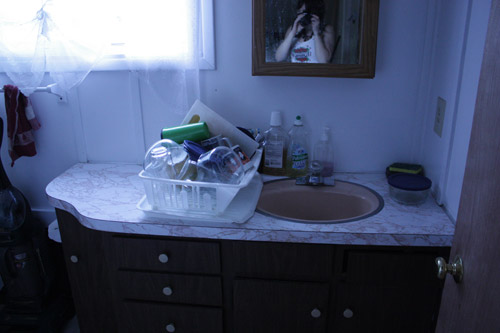In this image, we see a dimly lit bathroom featuring a dark-colored bathroom vanity with drawers and doors. The vanity is topped with a lighter-colored surface, possibly gray, which supports a pink rounded sink with a small chrome faucet. On the sink, there are bottles of mouthwash and dish soap. Next to the sink, inexplicably, there is a dish tray filled with various kitchen items, including cutting boards, plastic bowls, and a tumbler. A medicine cabinet is also present in the scene, and its mirror captures the reflection of the person taking the photograph, who appears to be a woman with dark hair wearing a white tank top. She holds a camera up to her face as she captures the unusual bathroom setup.